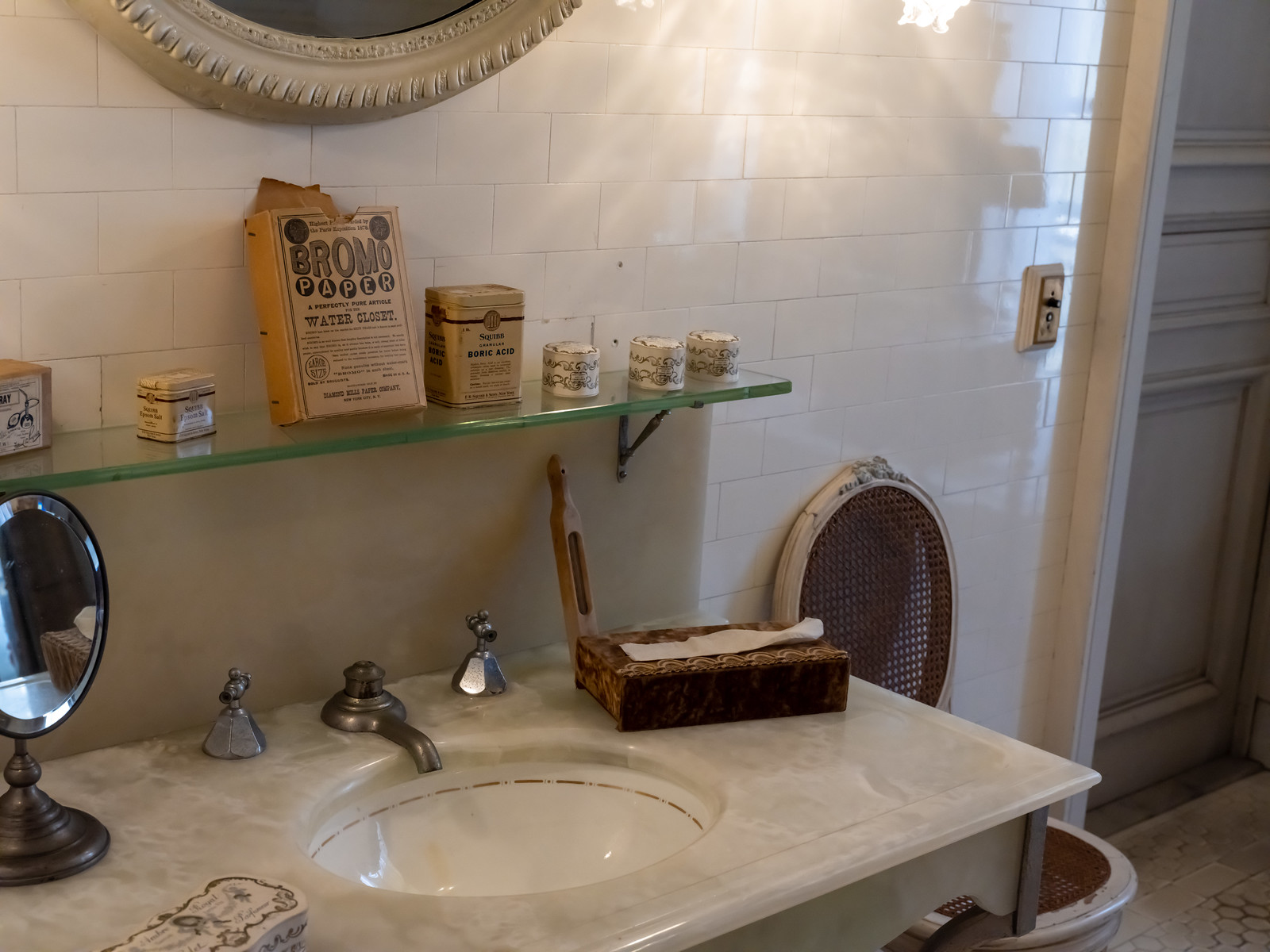This photograph captures a vintage bathroom with a distinctly old-fashioned charm. The walls are adorned with white tiles, creating a clean yet aged aesthetic. The door, painted an ecru shade, features intricate crown molding that adds a touch of elegance. The countertop, possibly crafted from quartz or marble, houses a rather unique toilet with a narrow rim and a woven lattice back instead of the usual ceramic top. The faucet is notably low, seemingly impractical for comfortable use.

On the countertop sits a mirror and a box of tissues, contributing to the room’s nostalgic feel. Above the sink, a shelf holds a striking collection of vintage items, including a box of Bromo paper and several small tins. Adding to the bathroom's ornate decor is an elaborate mirror positioned above the shelf, serving as a focal point that encapsulates the overall vintage atmosphere.